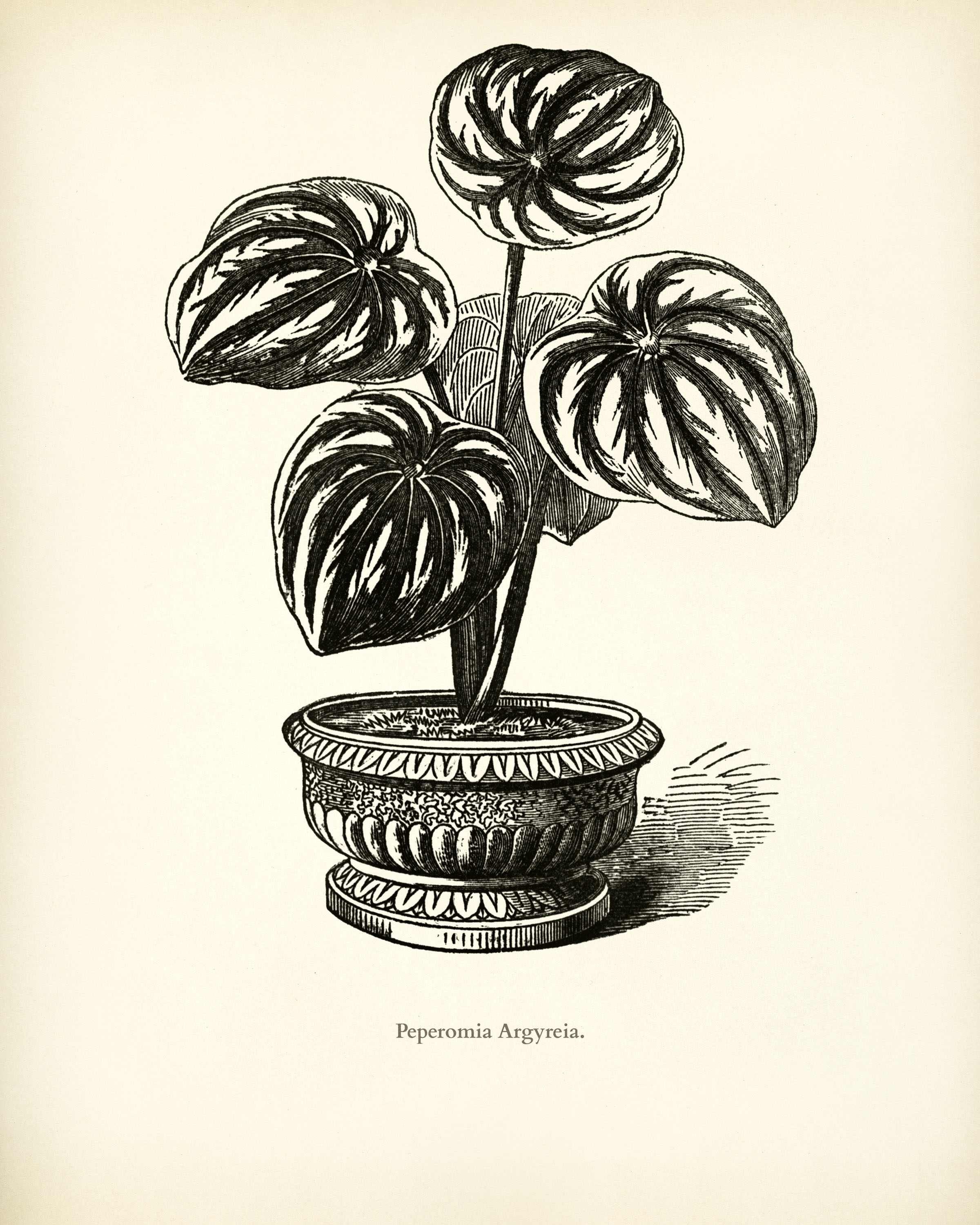The image is a detailed ink drawing of a potted plant on an aged, cream-colored background, reminiscent of old paper. The plant depicted is a Peperomia argyreia, clearly labeled at the bottom in black text as "P-E-P-E-R-O-M-I-A A-R-G-Y-R-E-I-A." The plant's pot features an intricate petal design along the rim and midsection and contains visible soil. The pot casts a shadow to the right, drawn using lines instead of traditional shading. The plant itself has approximately five large, heart-shaped leaves with pointed tips, resembling rhododendron or monstera leaves. These leaves exhibit long, vertical stripes that give them a somewhat pumpkin-like appearance. The drawing employs fine line work to add detail and shading to the leaves and the pot, contributing to an overall impression of meticulous craftsmanship.